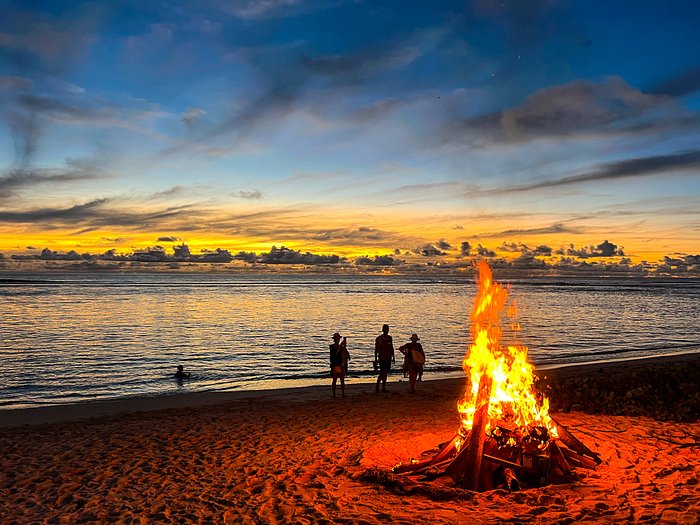This vibrant beach scene captures the essence of a tranquil evening at the shore. At the forefront, a lively bonfire illuminates the sand, casting a warm, reddish glow from the flickering flames as they rise from the stacked logs. The horizon features a breathtaking sunset, with a gradient of red, yellow, and blue colors painting the sky, accentuated by scattered clouds. The calm water gently laps the shore, where four people are enjoying the scene; one is in the water while three others stand close to the shoreline, their faces not clearly visible. They seem to be interacting or perhaps holding items like a chair or an umbrella. The play of light from the sunset and the fire creates a mesmerizing contrast against the growing darkness flanking either side of the image, completing this picturesque moment of a peaceful beach evening.